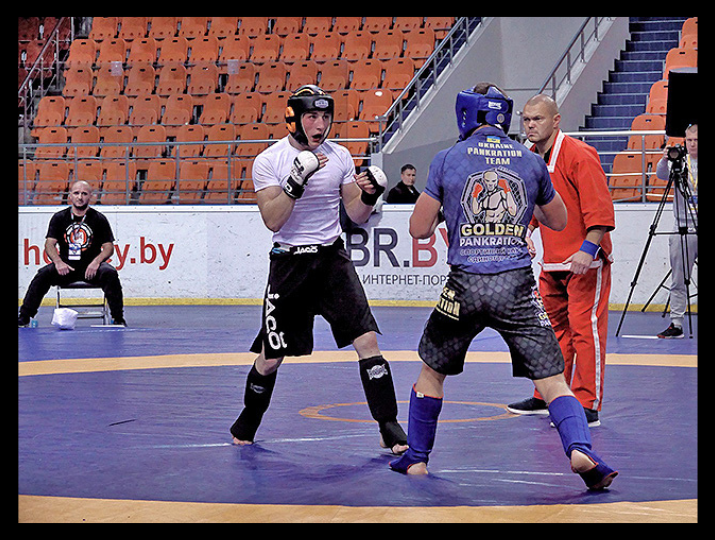The image captures an intense professional pankration fight between two white men on a blue wrestling mat in a stadium with empty stands featuring red and orange seats. The seated area is partially divided by a blue walkway, with someone standing in the middle of the division, and the stairs are also blue. One fighter, positioned on the left and facing us from his right side, is dressed in a white compression shirt, black shorts that have non-English white lettering, and black shin protectors with no shoes. He wears a black helmet with orange ear covers, MMA gloves that are white and black, and appears visibly tired with a mouth open and flushed cheeks. His opponent, facing away from us, sports a blue helmet, a blue shirt with the inscription "Golden Pankration," and a logo depicting a bald, muscular man with red gloves in a fighting stance. This second fighter also has black shorts with gray designs, blue shin covers, and no shoes, standing in a combat-ready stance. The referee in a red outfit with white stripes on the pants and black-and-white sneakers stands to the left, facing the fighters. In the background, a person on the far right is operating a camera on a stand, while another individual in black attire with a lanyard and pass sits on the far left, observing the match.